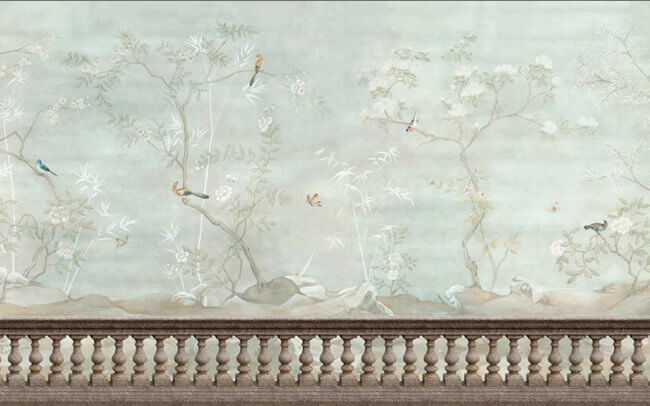The rectangular photograph captures an expansive open space dominated by a large, ornate stone or marble balcony railing in shades of gray and dark gray. Positioned behind this railing, a wall serves as the canvas for a sprawling, light-themed mural with a faint, pale green background. The mural, detailed in an almost oriental style, depicts a serene landscape of delicate, thin trees adorned with sparse white flowers at the ends of their branches. Scattered throughout the branches, various birds in different shapes and vibrant colors, including a blue jay, a woodpecker, and several red birds, add an element of lively diversity. The artwork extends across the entire wall, featuring elements such as tree limbs, some of which are prominently on the right side, and rocks on the ground. The base of the mural is bordered by repeating small pillars or silver stakes interspersed with a brown line above them, enhancing the sophisticated aesthetic of the scene.